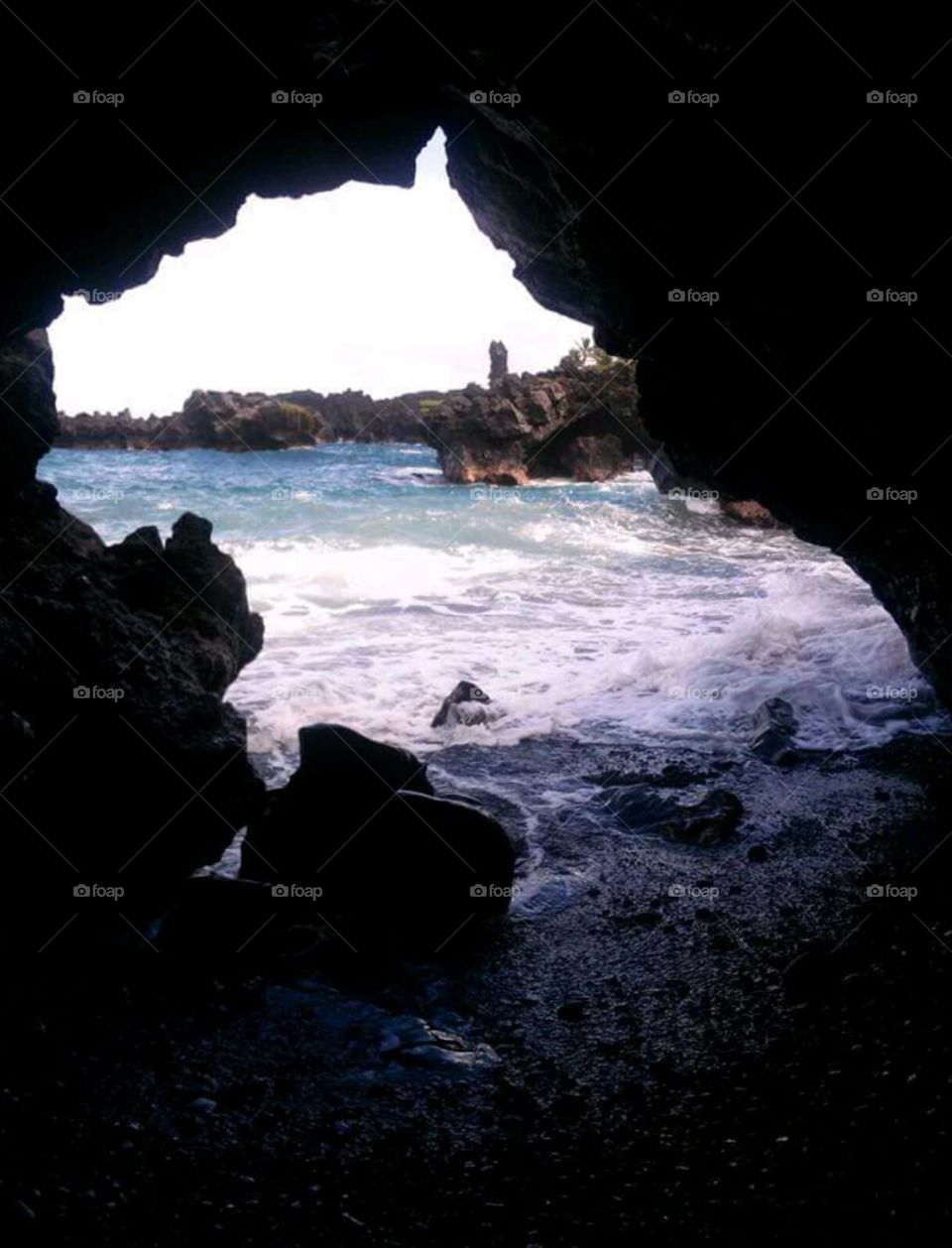This photograph captures a striking view from within a dark, cavernous cave, looking out onto the expansive ocean. The entrance to the cave is almost framed by an array of rocks, forming a rugged archway of dark gray and black. The cave interior is dimly lit, emphasizing the contrast with the bright scene outside. The foreground features the tide washing up against pebbles on the beach, creating white frothy surf. The ocean itself is a vivid blue, extending to a distant horizon where rocky formations or an island are perceptible, possibly adorned with patches of green foliage. The sky above the ocean is notably overcast, appearing as a washed-out white devoid of clear clouds. Watermarks labeled 'FOAP' along with a camera icon are distributed diagonally throughout the image, especially visible in the darker areas.